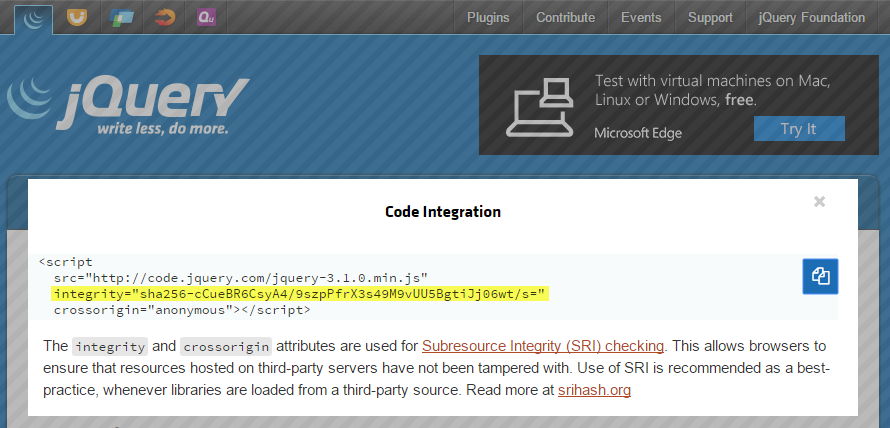This is a landscape-oriented screenshot of a website dedicated to coding or web design, distinguished by a diagonal white and black line pattern. The site is notably wider than it is tall. 

At the top, there is a horizontal black toolbar featuring diverse icons. The first icon is a logo comprising three crescent moon-like shapes decreasing in size, followed by an orange U-shape containing a white U, and several other indistinguishable symbols. To the right, clickable white-font labels read "Plugins," "Contribute," "Event," "Support," and "jQuery Foundation."

Below the toolbar, the jQuery logo (three crescent shapes alongside "jQuery" with a lowercase 'j' and capital 'Q') is prominently displayed, accompanied by the slogan "Write less, do more" in white text. Adjacent to this, a black box with white text reads, "Test virtual machines on Mac, Linux or Windows for free," featuring an illustration of a laptop, and inside its screen, a smaller laptop. A blue button labeled "Try it" is situated within this section.

Beneath this is a long, rectangular white box titled "Code Integration." Inside, a gray box contains a snippet of code with a highlighted yellow line, followed by an explanatory paragraph.

This detailed layout encompasses a structured, user-friendly interface focus on web development tools and resources.